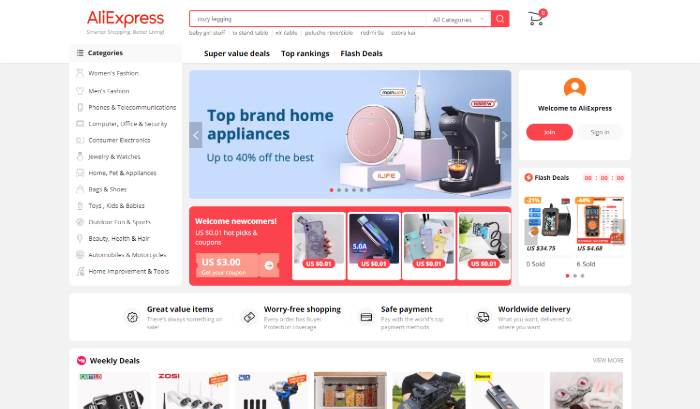This screenshot showcases the Aliexpress shopping website with a predominantly white background. On the left side of the page, there is a heading labeled 'Categories' which includes options like Women's Fashion, Men's Fashion, Jewelry, Bags and Shoes, Toys, among others. At the top of the screen is a prominent red rectangular search bar designed for product searches. The main section of the page displays various product images including a coffee maker, a mirror, and a water flosser. In the upper right-hand corner, there's an icon for the shopping cart to add items for online purchasing.